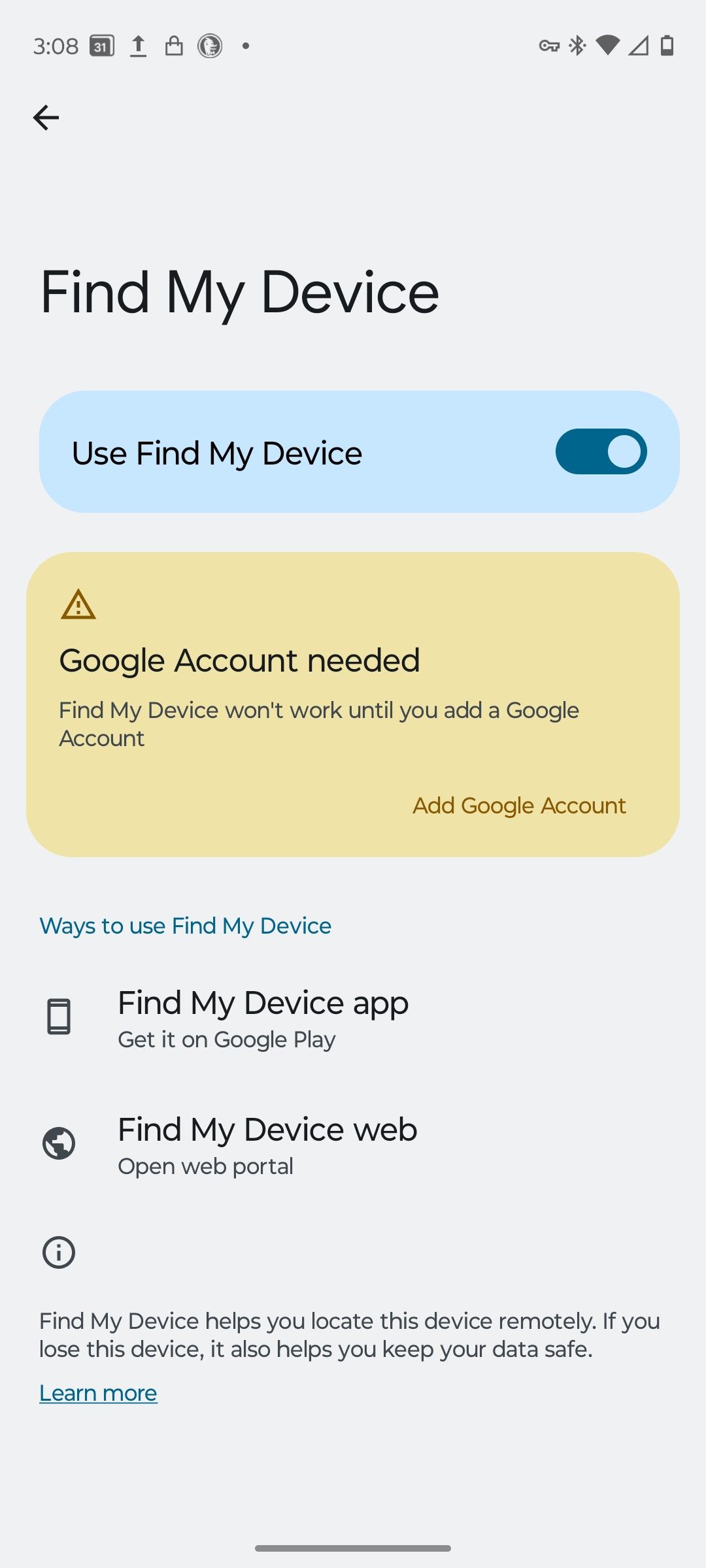**Detailed Caption for the Mobile Screenshot:**

The image depicts a vertical mobile screenshot with a gray background. In the top left corner, the time displayed is 3:08, along with several icons, including a calendar, an upload symbol, and an icon that resembles a shopping bag. On the top right, the battery icon shows approximately 20% remaining charge. Adjacent to the battery icon, there is a key symbol and a triangle pointing left.

Below these icons, black text reads "Find My Device." Immediately beneath this, a blue box with rounded corners highlights the message "Use Find My Device." To the right of the message is a slider, which is pushed all the way to the right. The slider is navy blue, while the small circle on the slider matches the light blue color of the surrounding box.

Directly under the blue box is a tan-colored box with the text "Google account needed." Inside this box, there is a warning triangle with an exclamation mark, followed by the message "Find My Device won't work until you add a Google account." At the bottom right of this box, brown text prompts the user to "Add a Google account."

Further down, in the gray section, there are options under "Ways to use Find My Device." The first option is "Find My Device app" with a prompt to get it on Google Play. The second option is "Find My Device web" with a prompt to open the web portal.

At the bottom of the screen, additional text explains, "Find My Device helps you locate this device remotely. If you lose this device, it also helps you keep your data safe," followed by a "Learn more" link.